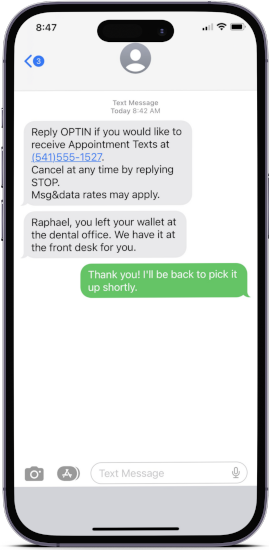The image depicts a highly detailed, edited mock-up featuring the iMessage app superimposed on an iPhone screen. The phone is oriented upright, with its screen facing the viewer. The iMessage interface is open, displaying a conversation with a user whose details and profile picture have been intentionally obscured for privacy.

Within the message thread, there are two incoming messages and one outgoing response. The first incoming message, received at 8:42 a.m., reads in all caps: "REPLY 'OPT-IN' IF YOU WOULD LIKE TO RECEIVE APPOINTMENT TEXTS AT 541-555-1527. CANCEL AT ANY TIME BY REPLYING 'STOP'. MSG AND DATA RATES MAY APPLY." The second incoming message is a more personalized note, stating: "Rafael, you left your wallet at the dental office. We have it at the front desk for you."

In response, the user sends a message saying: "Thank you, I'll be back to pick it up shortly."

The iMessage interface is clearly visible, complete with its characteristic design elements. In the bottom left-hand corner, there is a camera icon for sending photos, alongside a button to access various apps. Additionally, there is a text input field, as well as an option to record or dictate an audio message.